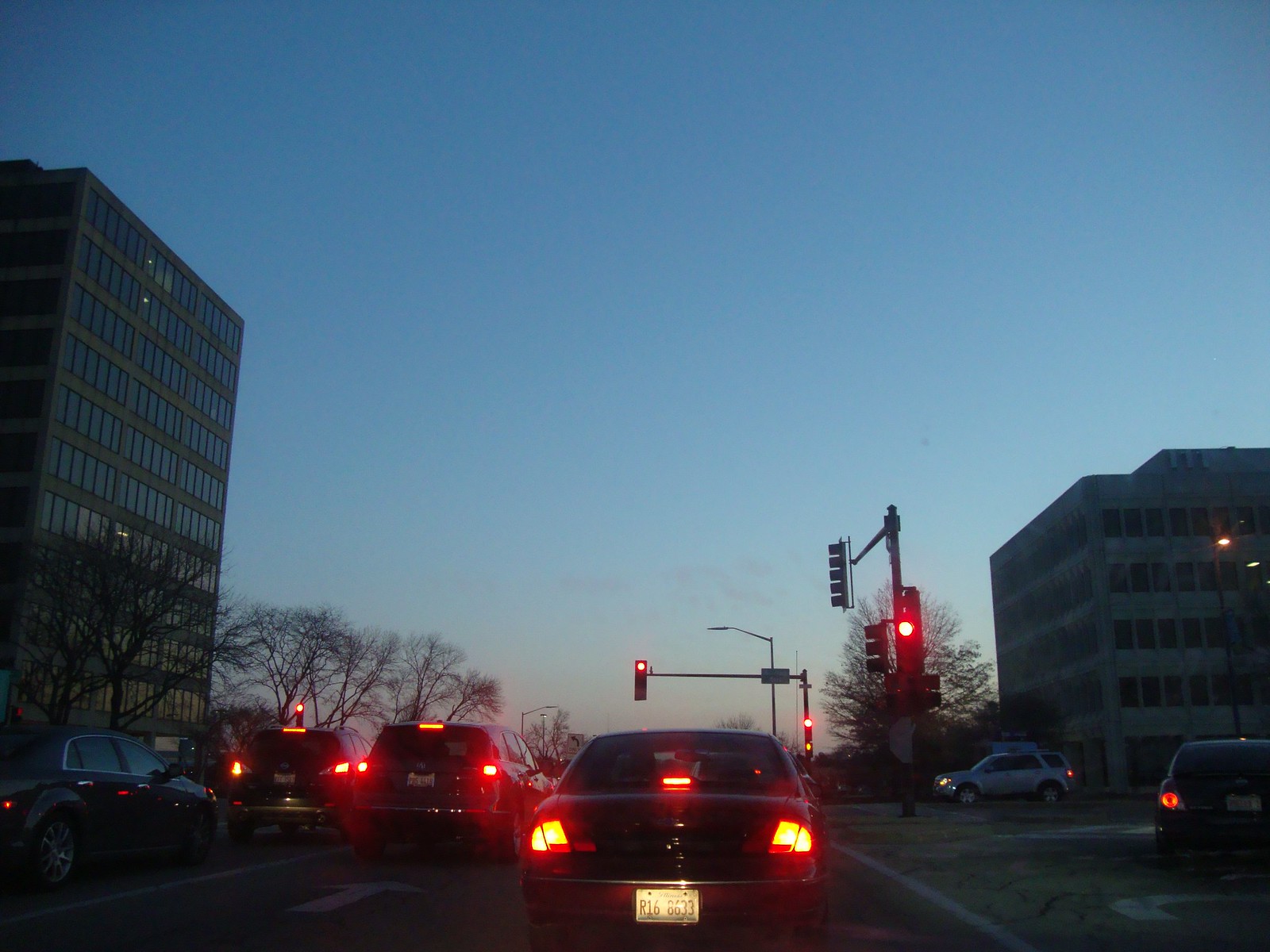The photograph captures a serene sunset moment from the perspective of a car on a street, facing a red traffic light. Ahead, five cars are waiting at the stoplight, their brake lights glowing softly in the dimming light. The sky exhibits a captivating ombre effect, with a gentle orange hue near the horizon gradually blending into a darker blue as it ascends. To the left of the scene stands a tall, approximately ten-story building with numerous windows, while on the right, there's a shorter five-story building, also adorned with many windows. A sizable tree is present on the left side near the vehicles, and another large tree is visible on the right, in front of a white SUV. Overall, the calm intersection, dotted with buildings and trees, captures the essence of a typical urban evening transitioning into night.